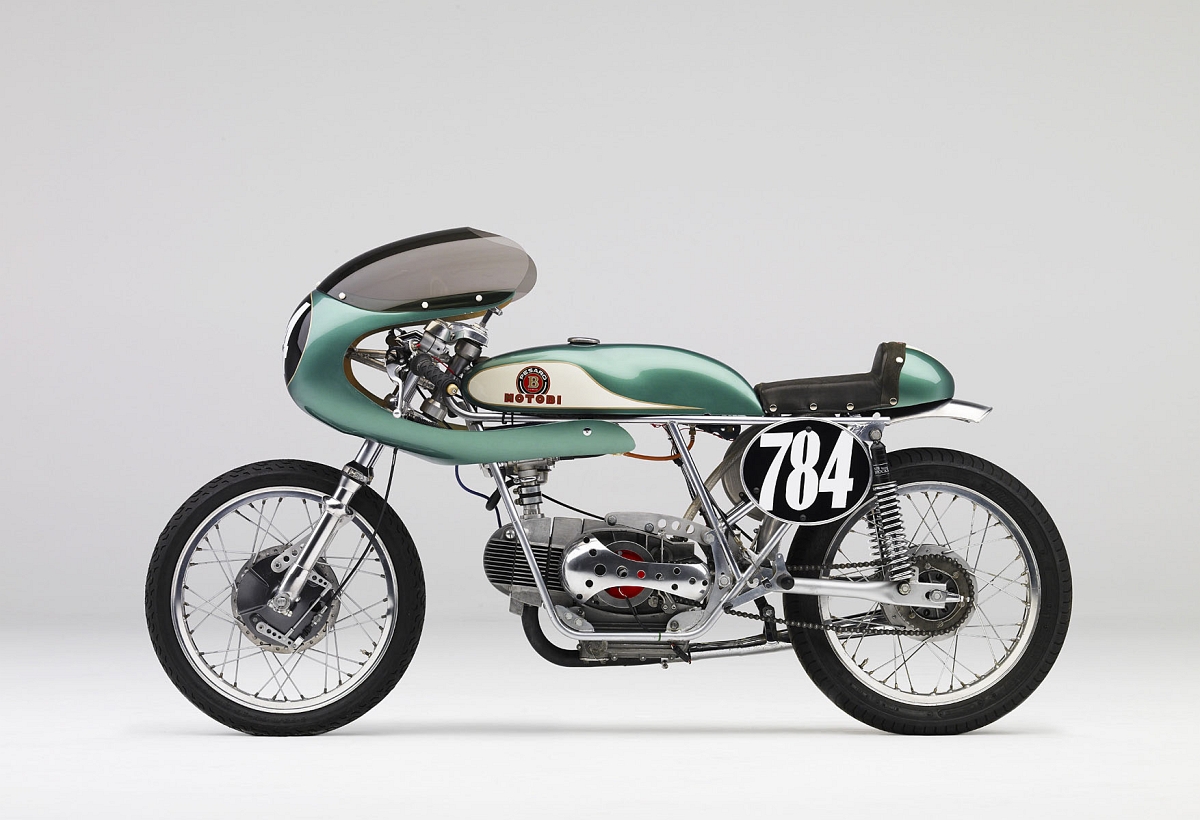The image depicts a distinctive motorcycle set against a stark white background, likely photographed in a studio. The motorcycle, facing left, boasts a retro-futuristic design, reminiscent of a 1950s vision of the future. Its body is predominantly metallic jade with a cream panel. The text "Motobi" in red is emblazoned on the body, alongside a unique circular logo featuring a "B". A notable feature is the number "784" prominently displayed near the back wheel in a black circle with white font. The back wheel is slightly thicker than the front, and both tires are studded with distinctive spikes. The engine, located below the main body, is a gleaming silver, adding to the machine's intricate mechanical appeal. A dusty grey windscreen extends from the front, yet the absence of handles hints at a design that blends both historic and futuristic elements.